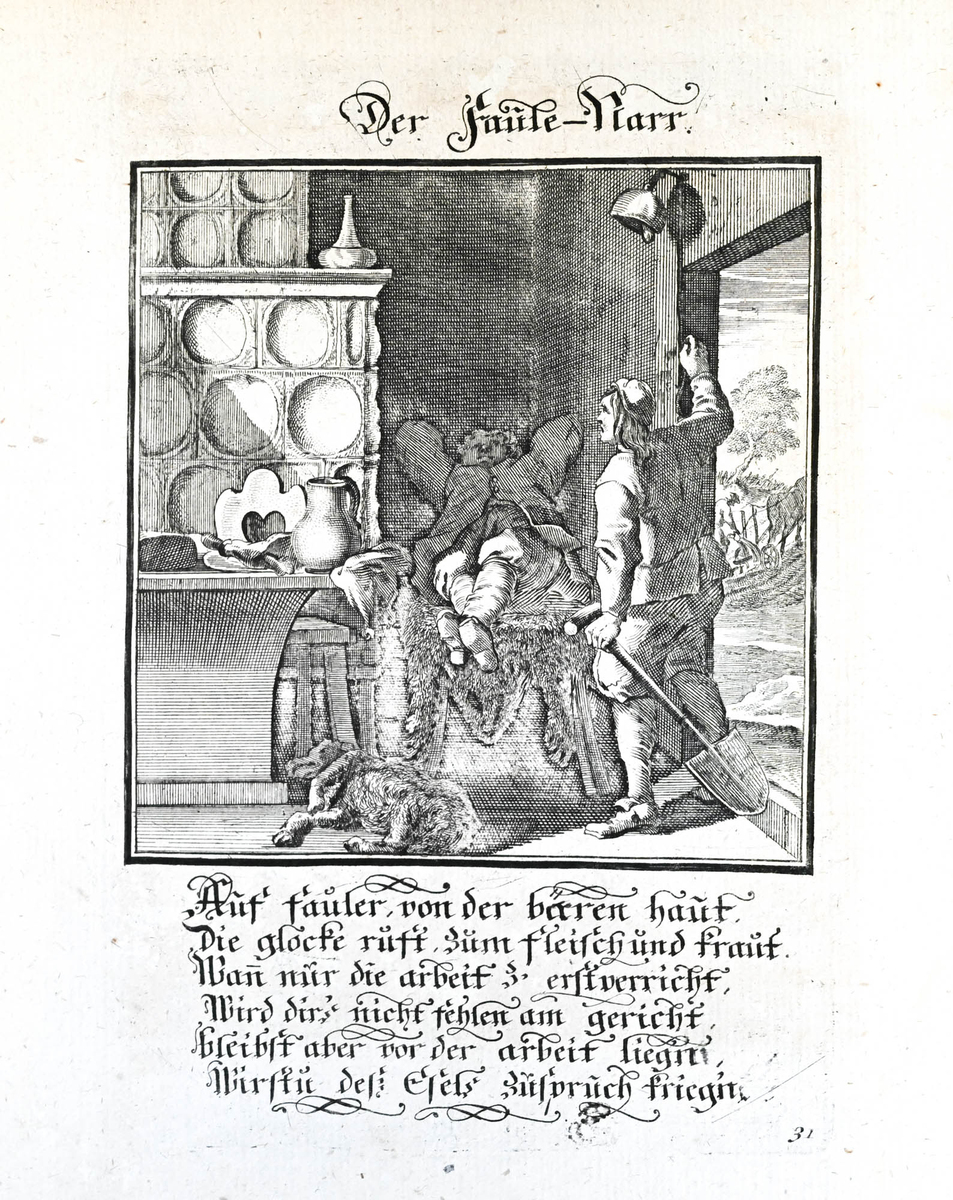This black and white illustration, printed on white paper, presents an intricately detailed scene with elaborate German script and specific elements of what seems to be a colonial or old-world setting. Centrally, it depicts a man reclining on a fur-covered chair, mouth agape in deep sleep, while a loyal dog slumbers on the floor at his feet. To the side, a worker dressed in white attire stands at a doorway, clutching a spade in his left hand and reaching up to ring a bell mounted above the door with his right. In the background, stacks of barrels suggest the room might be part of a brewery or farm outbuilding, reinforced by the presence of a jug and various items on a nearby cabinet. Equally eye-catching is the elaborate script text, featuring the German phrase "Der Fahrt Paar" at the top, and a page number, 31, at the bottom right corner. The countryside outside the establishment, dotted with trees and a horse, completes the picturesque scene.